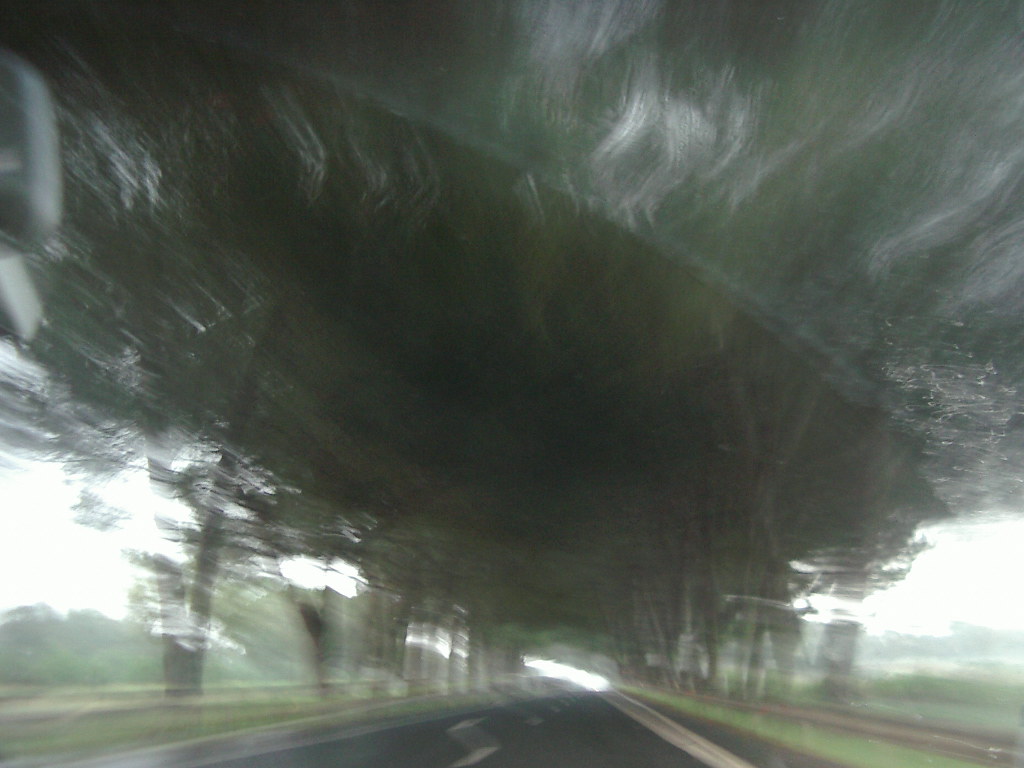The image, most likely captured from a moving car through a windshield, is highly blurry and distorted. A significant portion of the frame, approximately 75%, is dominated by a green haze formed by blurred treetops with thin trunks, suggesting the presence of surrounding vegetation. The asphalt road is prominently featured, but its appearance is greatly affected by the motion, resulting in wavy and misaligned center dashes that fail to form a coherent line. On the right side of the image, a rusty-looking guardrail is visible, adding an element of structure amidst the chaos of the blur. In the distance, a landscape of grassy fields with scattered trees can be discerned, though it too is affected by the motion-induced blur. The overall impression is one of speed and motion, with the natural scenery melding into a green, vegetative blur.